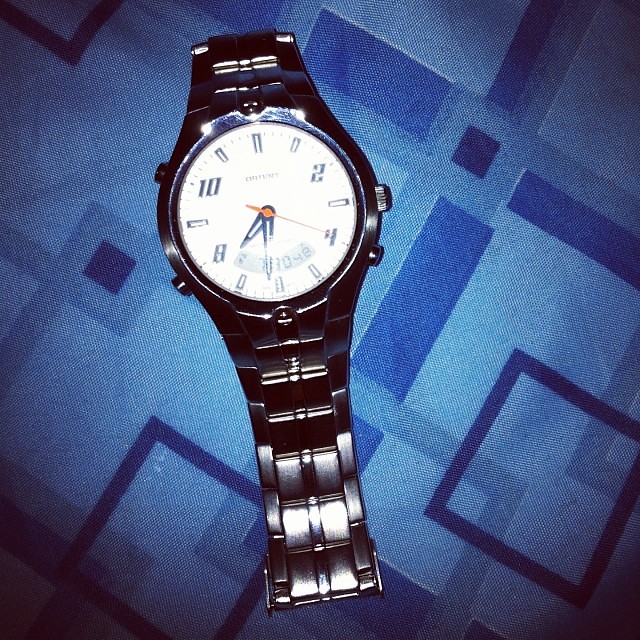This highly detailed photograph captures a metal wristwatch lying on a surface that features an intricate blue pattern. The surface, which could be a carpet or a bedspread, displays a design of varying blue hues, with small dark blue squares surrounded by lighter blue lines and larger dark blue squares interspersed throughout. The watch, entirely crafted from metal, showcases a band composed of interlocking metal links that extend seamlessly around from the clasp to the face. The watch face is protected by a glass plate, beneath which lies a white dial with black hour and minute hands, currently indicating the time as 7:32.